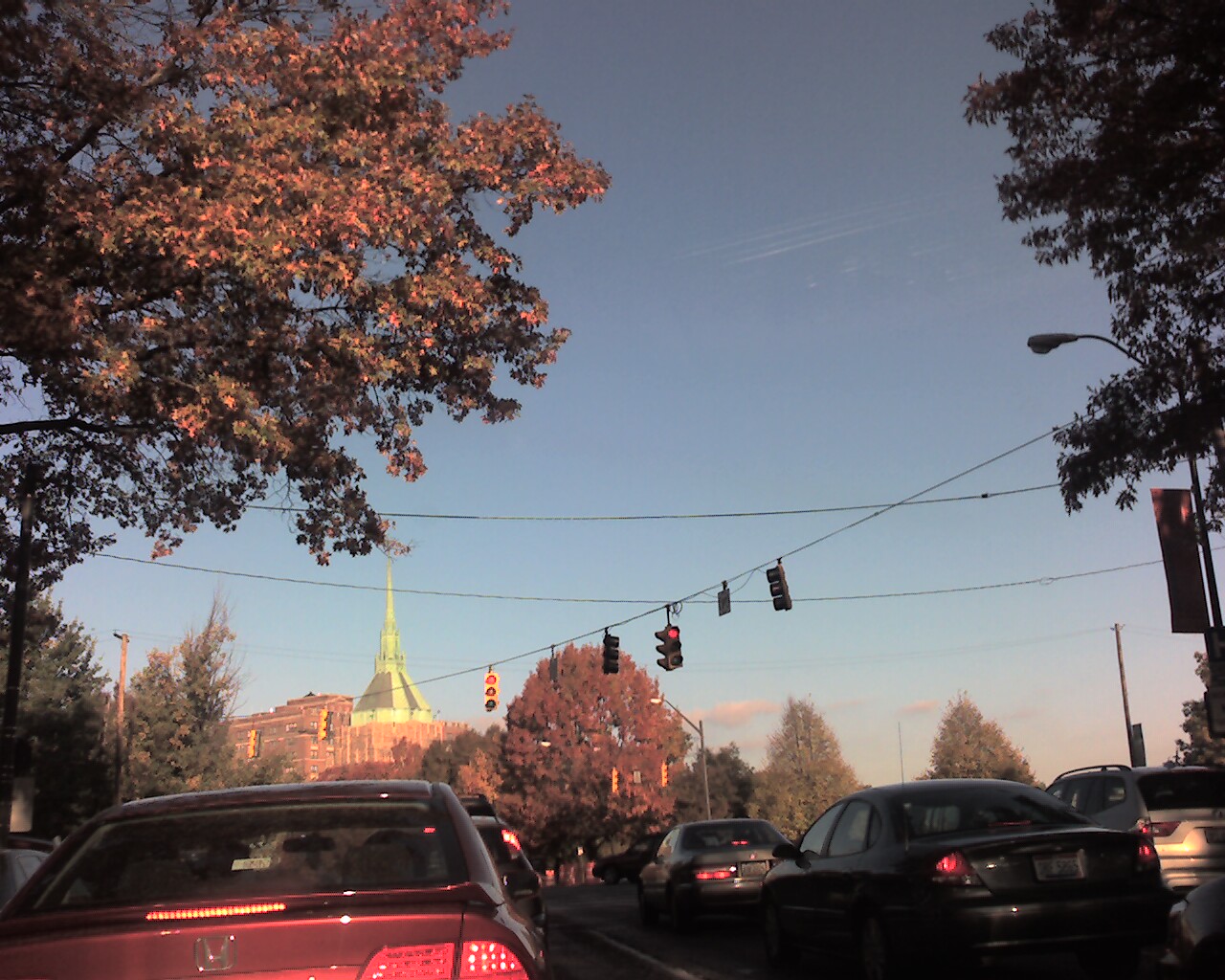This image, captured from inside a car stuck in traffic, showcases a congested intersection on a clear, sunny day. In the lower left corner, a red sedan coupe is prominently visible, followed by a line of vehicles ahead. Directly ahead, there is a black four-door sedan, and further in front of it, a gold four-door sedan. Both sedans sit close together, aligning within their lanes. The intersection is controlled by two traffic lights directed towards the viewer, both displaying red signals, and two additional lights facing other directions. The bright blue, cloudless sky creates a sharp contrast with the verdant deciduous trees, which display a mix of green and brown leaves in the upper corners of the image. In the distance to the left, a church steeple rises above the treetops, adding a touch of architectural interest to the serene outdoors scene.